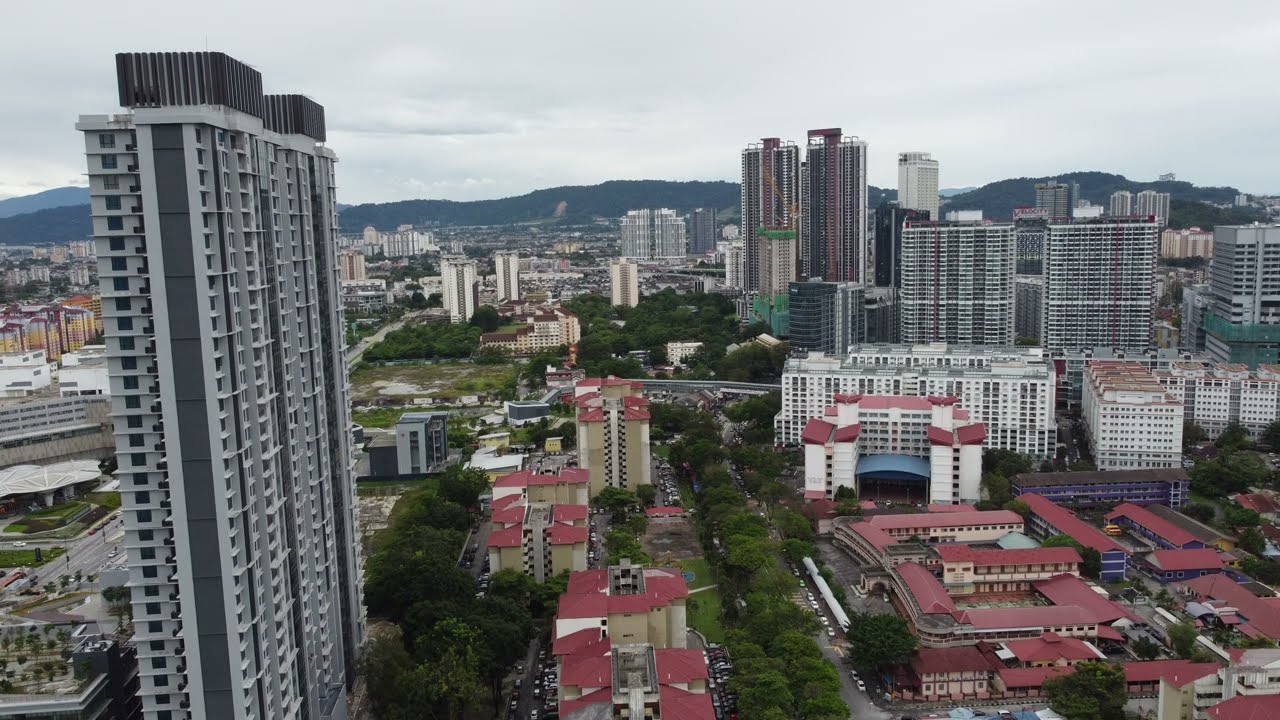This aerial color photograph, depicting a detailed cityscape in landscape orientation, captures a bustling small city from above during the middle of the day. The left side of the image prominently features a large, high-rise building with a gray concrete finish and black vertical structures on its roof. Adjacent to this high-rise are several smaller buildings, distinguished by their red tile roofs, dispersed among lush greenery, including trees and bushes. These shorter, more residential or commercial buildings are interspersed throughout a green belt that stretches through the center of the image. As one looks further right and towards the background, taller multi-story buildings emerge, characterized by their bland facade of floors and windows, varying in shades of gray and brown. 

Towards the horizon, the image showcases a distant mountain range or low hills in dark blue tones extending from left to right, under a sky densely covered with white and gray clouds. The overall setting appears to be outdoors, under considerable cloud cover, giving the photograph a somewhat muted yet realistic representation. The cityscape is comprehensive with details of the structures' varying heights and designs, scattered in a way that no single element dominates the foreground, providing a balanced and immersive view of the metropolitan environment teeming with architectural diversity alongside strands of greenery.